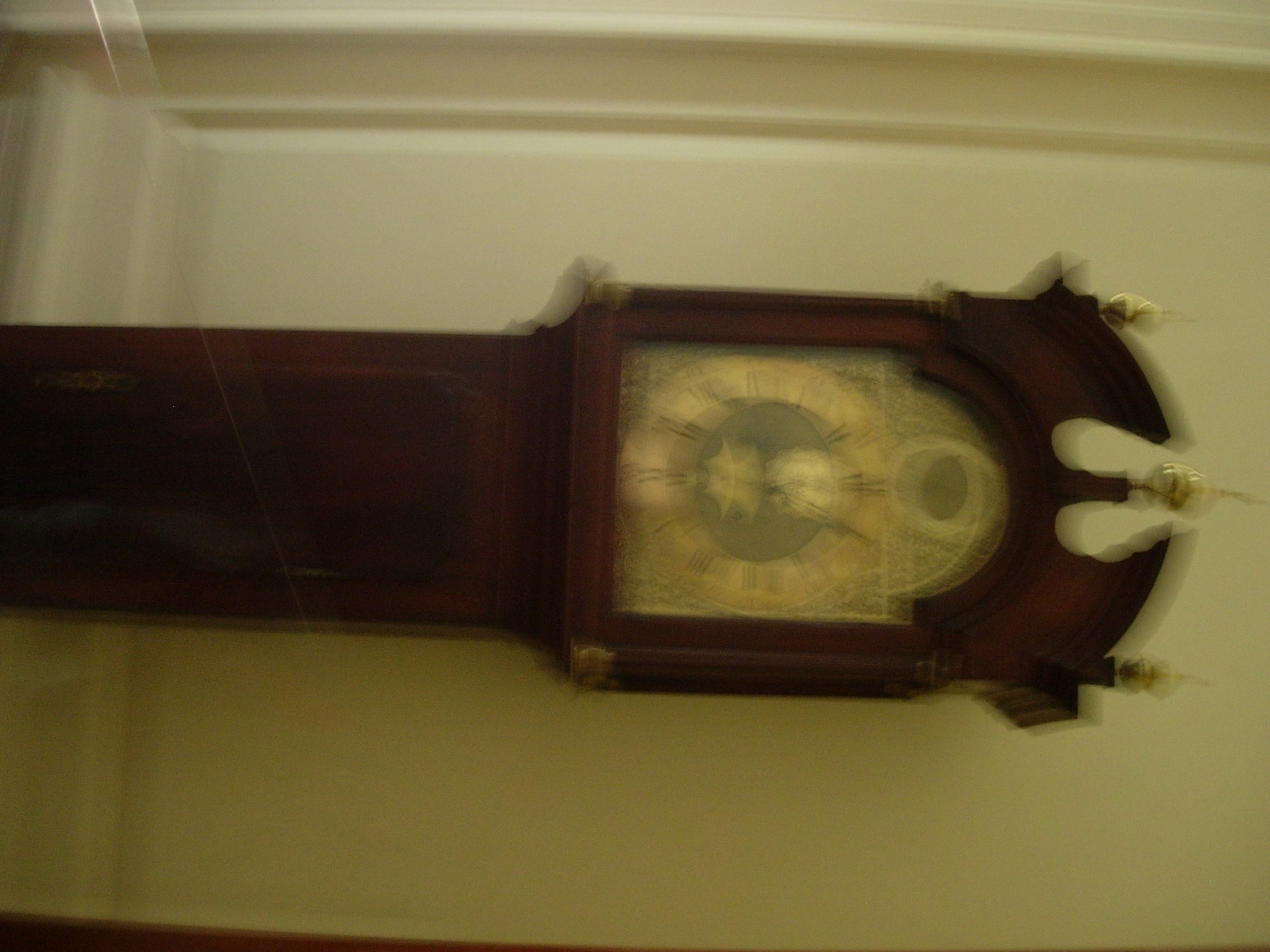The image is a very blurry photograph of a large, ornate, brown grandfather clock positioned against a cream-colored wainscoted wooden wall. The photograph is oriented sideways, with the top of the clock pointing to the right side of the image. The clock has a wooden frame that displays intricate craftsmanship, and its face, which appears to be a goldish or creamy light brown, features Roman numerals. There are gold or brass ornamentations around the face and at the crown of the clock. The base of the clock gets cut off before the bottom can be seen, and on the left side of the sideways photograph, part of the clock's stand and a handle are visible amidst the blur. The overall appearance of the clock suggests it is made from a deep cherry wood or mahogany, contributing to its vintage, grand design.